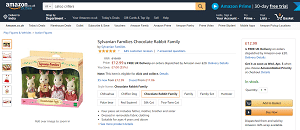This is a detailed screenshot of a product page on the Amazon website. At the top, a black navigation bar displays the white Amazon logo on the left, with the yellow "Prime" label adjacent to it. Next to this is the "All" drop-down menu for category selection and a prominent central search bar, flanked by a yellow search button with a magnifying glass icon. To the right, the bar offers promotional links, account options, order history, and a shopping cart icon with a numerical indicator for the items added.

Below the navigation bar, on a white background, is a product image featuring a toy set of four white rabbits housed in a tan box. The rabbit family includes a mother in a pink dress with a white apron, a father in brown pants paired with a vest, and two children, a boy and a girl. Additional frames to the left provide various angles and close-ups of the product. To the right of the main image, there is a comprehensive product description including features, star rating, and price information. On the far right side of the page, a purchasing box presents options to add the item to the basket or save it for later, alongside the current price.